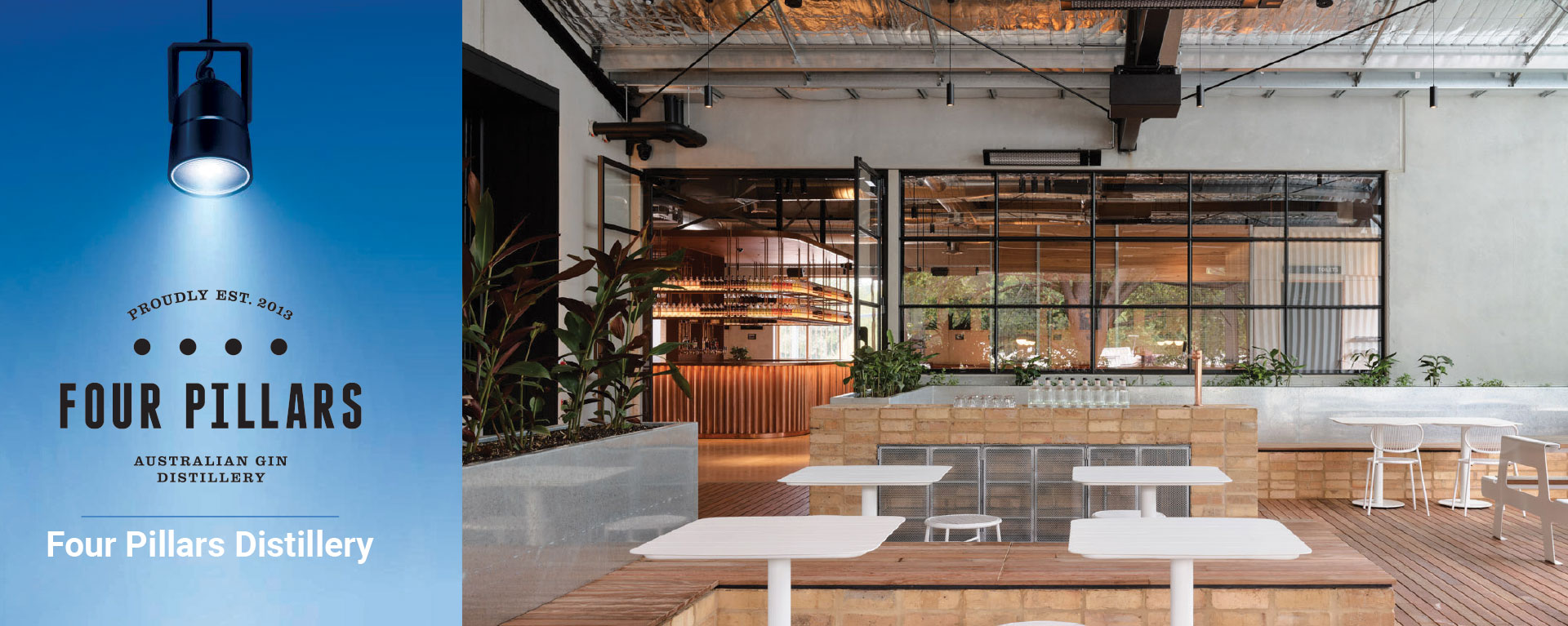This is an advertisement for the Four Pillars Distillery, established in 2013. The ad is horizontally rectangular, with the left third dedicated to a blue background spotlighted from above. In this section, the text "Proudly EST. 2013" is highlighted in black uppercase letters, arched above four black dots. Below, larger black uppercase letters spell out “FOUR PILLARS,” followed by smaller black text stating “Australian Gin Distillery.” A thin blue line separates this from the final line, which in white letters reads “Four Pillars Distillery.”

On the right side of the ad is a photograph showcasing the distillery’s modern, open-concept interior. The space is predominantly white with high ceilings and a clean, elegant appearance. A large, multi-paneled window with brown grid framing dominates the background, allowing in ample natural light. Below the window, a well-stocked bar with wooden trim and hanging glasses can be seen. 

The seating area includes multiple small white tables and white stools, with additional seating provided by wooden benches set atop tan-colored brick bases. Green potted plants add touches of color, with a particularly large white planter box on the left side overflowing with tall greenery. The overall effect is of a bright, sophisticated, and welcoming environment, perfect for enjoying gin and socializing.